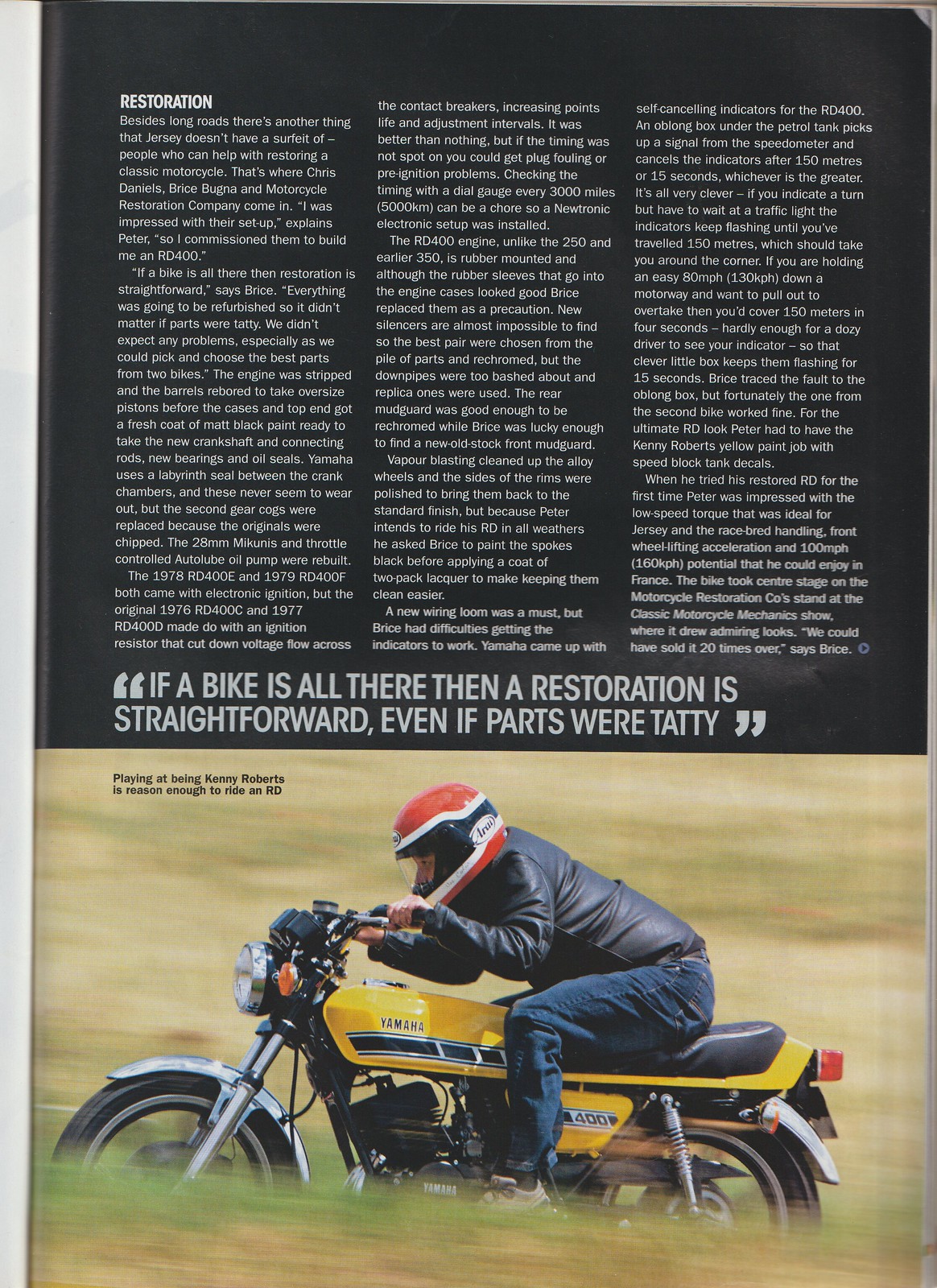The magazine page features a visually striking layout with a stark black background and three long columns of white text at the top, labelled "Restoration." The article delves into the merits of motorcycle restoration, including a quote, "If a bike is all there, then a restoration is straightforward, even if parts were tatty." 

Beneath the text, a large, vibrant photograph captures the essence of the content. The image showcases a man riding a yellow Yamaha motorcycle with a black leather seat and a prominent black stripe along the tank. The rider, equipped for speed, dons a red, white, and black helmet, a black leather jacket, dark denim jeans, and gray shoes, accentuating his determined posture as he leans into the handlebars. The dynamic scene unfolds against a lush, grassy landscape, with a green hill serving as a scenic backdrop. The photograph's caption, "Playing at being Kenny Roberts is reason enough to ride an RD," underscores the thrill and allure of embodying a legendary motorcyclist.